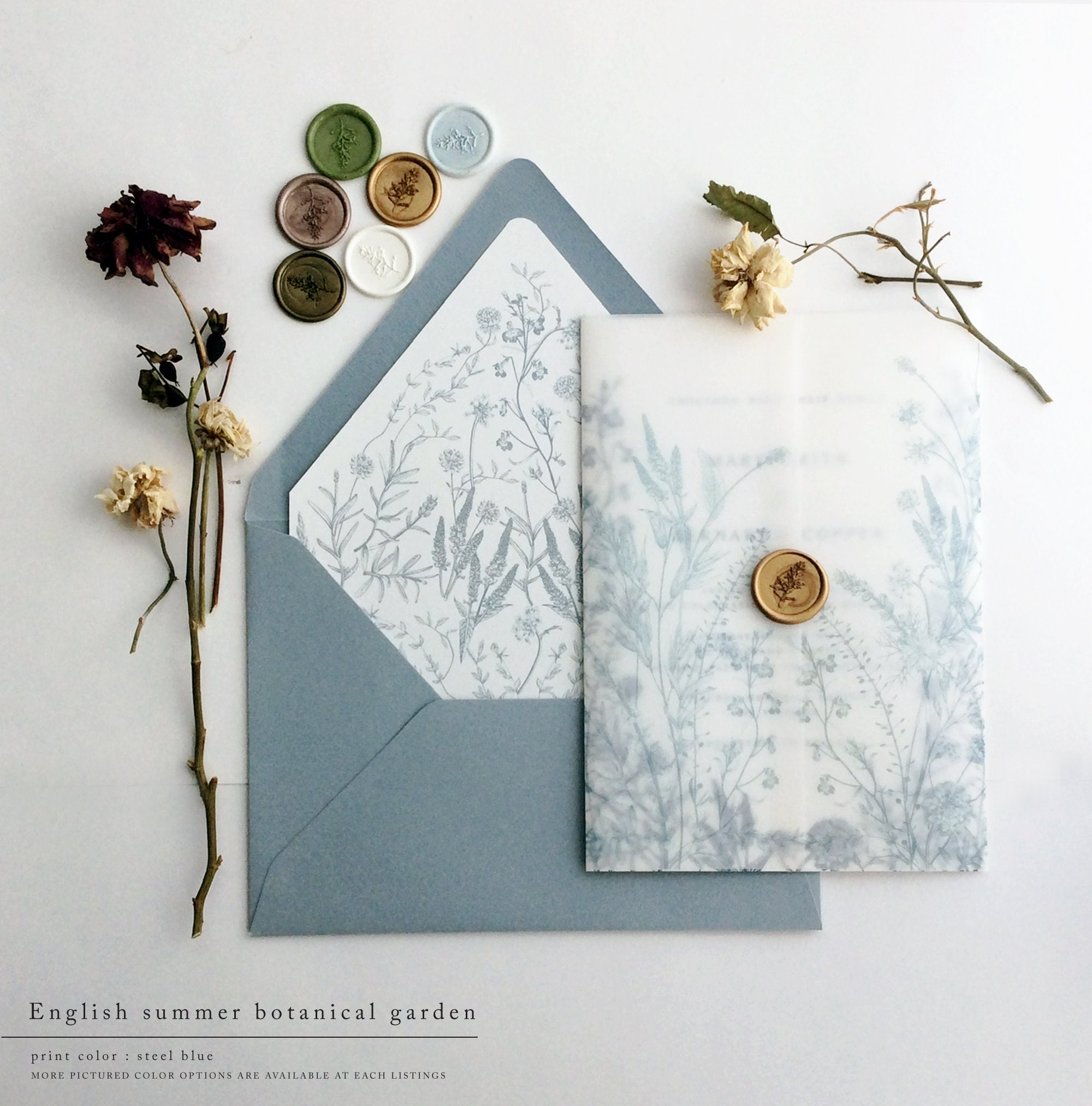This vertical rectangular image showcases an elegant stationery set titled "English Summer Botanical Garden" in the bottom corner. At the forefront is an open gray envelope, lined with white paper featuring a steel blue design, which matches the note card intended for the envelope. Accompanying the set are several colored wax seals or coin-like discs, including green, purple, gold, white, copper, and steel blue, each with unique inscriptions. Scattered throughout the image are various dried flowers and twigs, adding a rustic charm. The print color is noted as steel blue, with additional color options available.